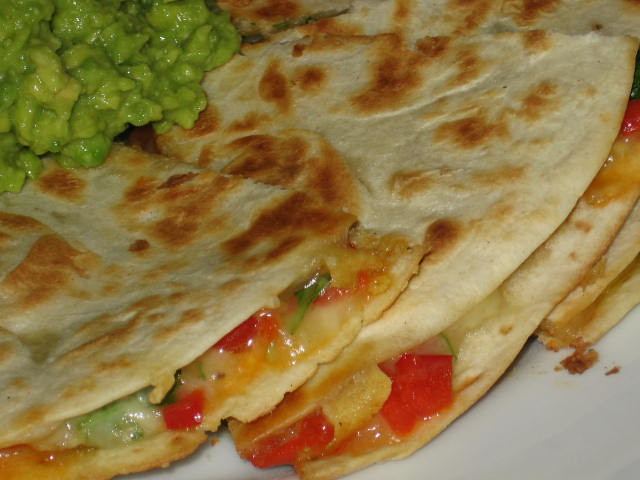This is an extreme close-up color photograph of three beautifully browned, toasted quesadillas on a barely visible white ceramic plate. The quesadillas are layered on top of each other, showcasing their toasty, skillet-fried exterior. Inside, the melted cheese oozes out, revealing a combination of both white and orange cheeses, likely Swiss and cheddar. Alongside the cheese, small cubes of tomato and perhaps some salsa add vibrant color. A generous portion of chunky, green guacamole sits atop the quesadillas in the upper left corner, its moist texture contrasting with the crispy quesadillas. In the upper right corner, a bit of tomato peeks out, hinting at the delicious filling within.